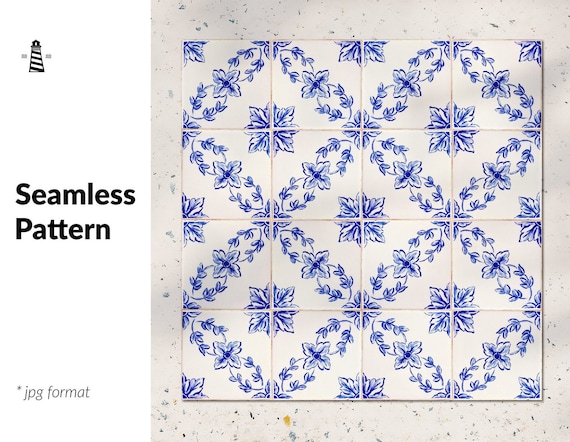This photo captures a seamless pattern in a JPEG format, featuring a vivid, repeating design reminiscent of a jigsaw puzzle or intricate floral quilt. The entire pattern is organized in sections arranged in a grid of four rows and four columns, each section forming a square. These squares collectively create an infinity or the number eight shape due to the interlocking design. At the center of each set of four squares, there is a detailed blue-floral motif, which further ties into the interconnected theme with blue vines extending through the pattern. 

The design is bordered by a cream-colored frame with wiggly lines, adding a hand-drawn aesthetic. Within each square section, the blue flowers and vines form a secondary square at the intersections where the rows and columns meet. The pattern sits atop a white countertop speckled with black sparkles, adding a textured backdrop to the photo. The meticulous arrangement and the interwoven floral motifs are suggestive of traditional China plate designs or elegant wallpaper, but here, they come together to form a quilt-like composition.